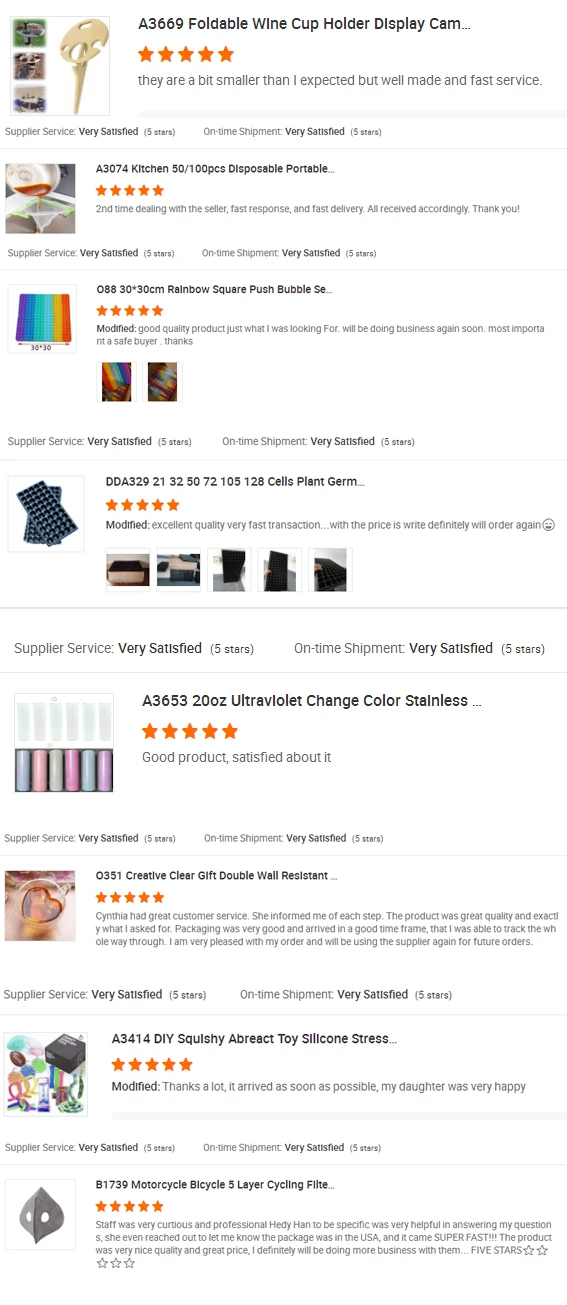The image depicts a person browsing an online shopping app on their smartphone. At the top of the screen, there’s a product listing for a "Foldable Wine Cup Holder Display Cam," which is rated five stars. The customer review mentions, "A bit smaller than I expected, but well made and fast service." Beneath this item, there is a "Kitchen Disposable Portable" listed, accompanied by a review stating, "Second time dealing with the seller, fast response, fast delivery, all received accordingly, thank you."

Scrolling further down, the user encounters a "Rainbow Square Push Bubble Set," with a reviewer praising, "Good quality product, just what I was looking for, will be doing business again soon, most important, a safe buyer, thanks." The page continues to display various items, including a "Cells Plant Germ," an "Ultraviolet Change Color Stainless," and a "Creative Clear Gift Double Wall Resistant."

As the user scrolls down, more products are visible, such as a "DIY Squishy Abrect Toy Silicone Stress" and a "Motorcycle, Bicycle, Five Layer Cycling Filter" at the bottom of the page. The listings are presented with product images, names, and customer reviews, providing insight into the shopping experience and consumer satisfaction.